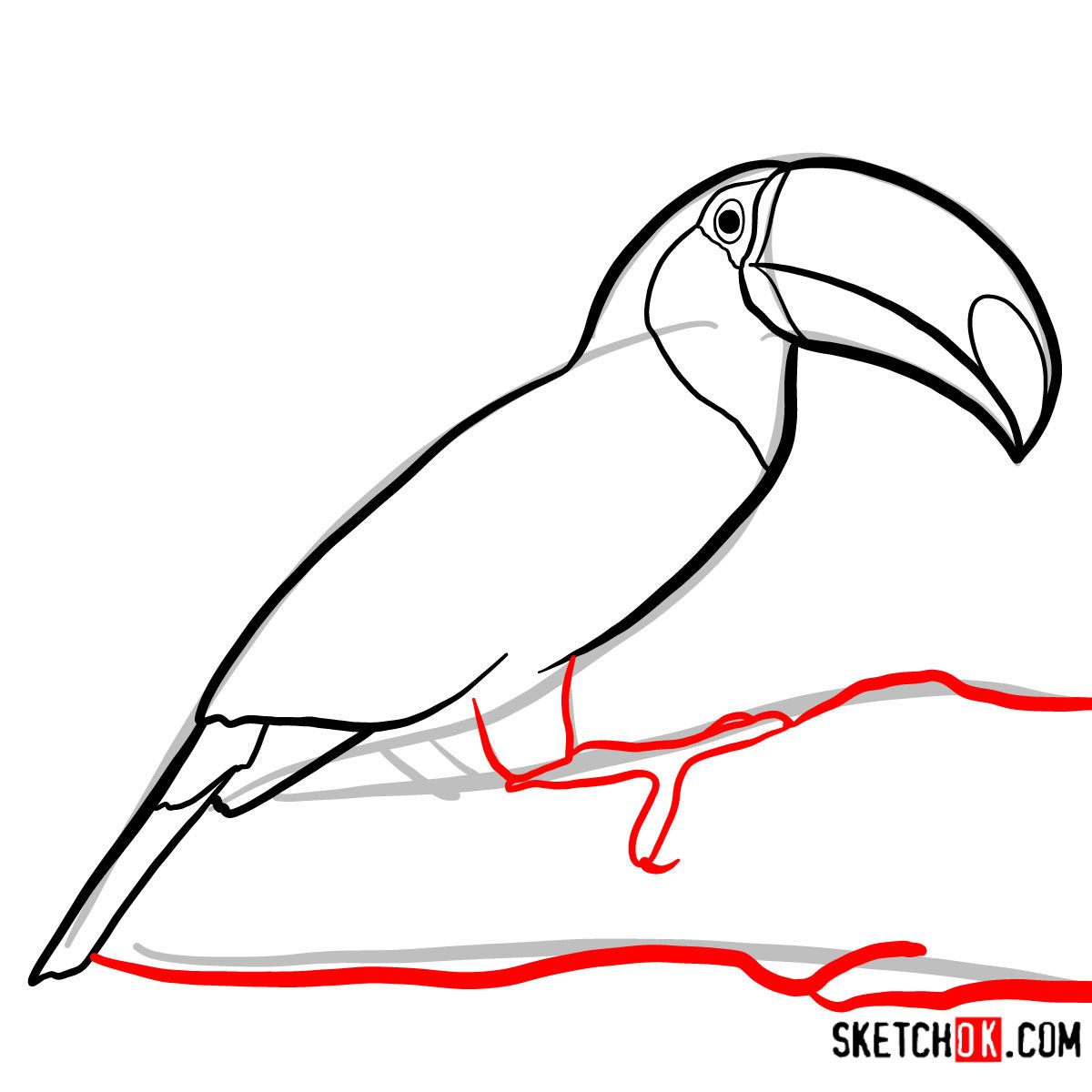This image is a detailed digital illustration of a toucan, a tropical bird native to the jungles of South America, often remembered from a 70s and 80s cereal commercial. Predominantly black and white, the sketch features the toucan standing upright on a branch, facing right. The bird's body is outlined in medium-width black pen, with red used to highlight the legs, feet, and some branches. There are also touches of gray on parts of the tail. The simple backdrop, featuring a single branch line, leaves the white background largely untouched. The bottom right corner bears the text "sketchok.com," indicating the source of the artwork.